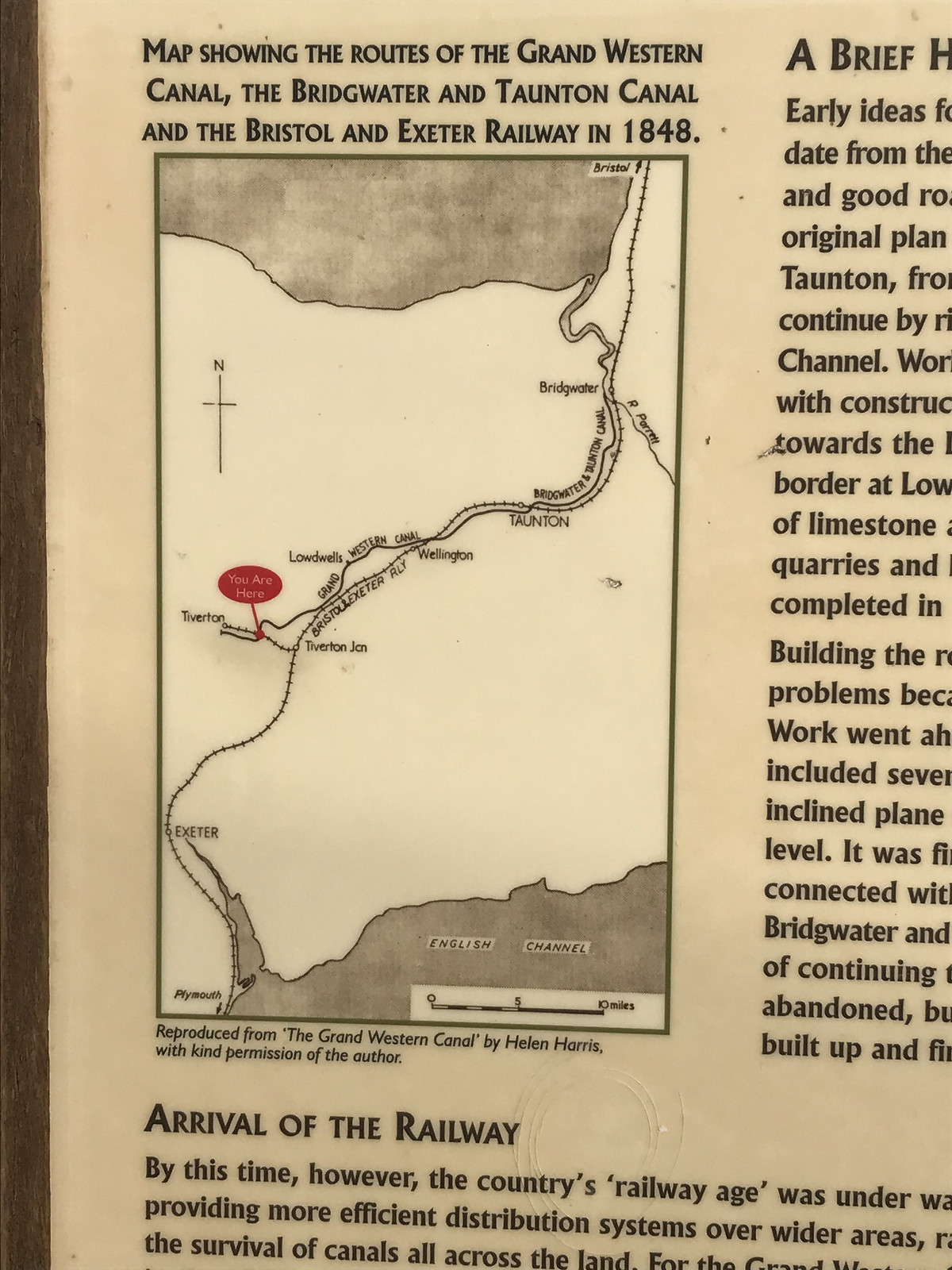This black and white image has an aged appearance reminiscent of an old newspaper or a historical booklet, characterized by a sepia tone and faded white pages. Dominating the image is a detailed map showing the routes of the Grand Western Canal, the Bridgewater and Taunton Canal, and the Bristol and Exeter Railway in 1848. Accompanying this map is clear, legible black text offering historical context. At the top, there's a prominent title reading "Map showing the routes of the Grand Western Canal, the Bridgewater and Taunton Canal, and the Bristol and Exeter Railway in 1848." In the center of the map, a red dot marked "you are here" highlights a specific location among the intricate network of canals and railway lines. To the right of the map, more text provides additional context, possibly titled "A brief history," although the word 'history' is partially obscured. At the bottom of the page, another heading in larger, darker print reads "Arrival of the Railway," followed by more information that, unfortunately, trails off and becomes unreadable. The overall impression is of a clear, perhaps zoomed-in, detailed page that might belong to an informational plaque, a billboard, or an educational display in a visitor center.